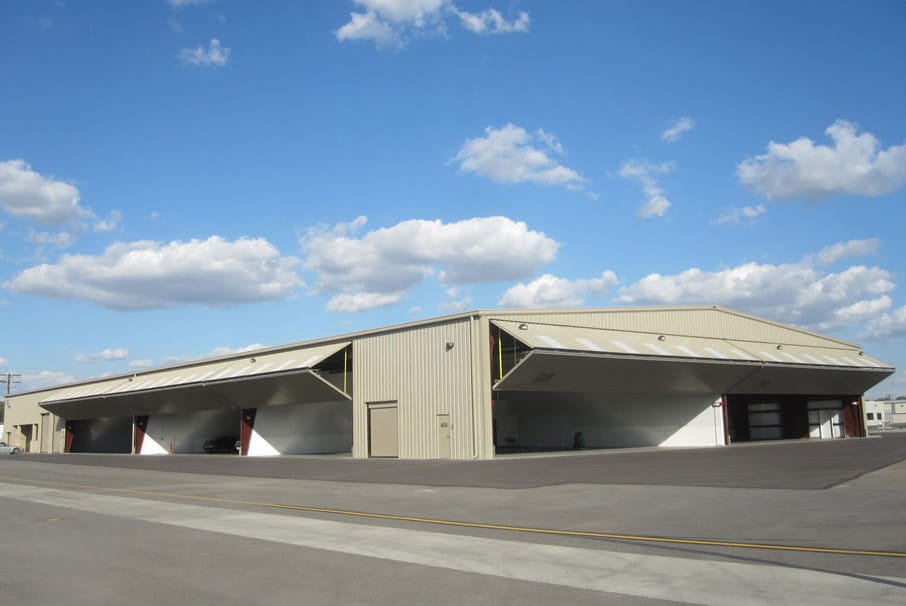This color photograph, in landscape orientation, showcases an airport hangar or warehouse facility under a blue sky dotted with white, puffy clouds. The building, constructed of vertical corrugated metal painted in a light green hue, features a large door on the right side that retracts upwards, partially revealing the interior. The left side also has a sizable door, fully open, exposing three interior bays painted in white and red. Within this open section, a black car is parked in one of the spaces to the left. Adjacent to the building, a white car is parked on the asphalt lot, which is marked with yellow lines running across it. The predominant external colors of the structure appear to be yellowish or brownish, complementing the industrial aesthetic of the scene.